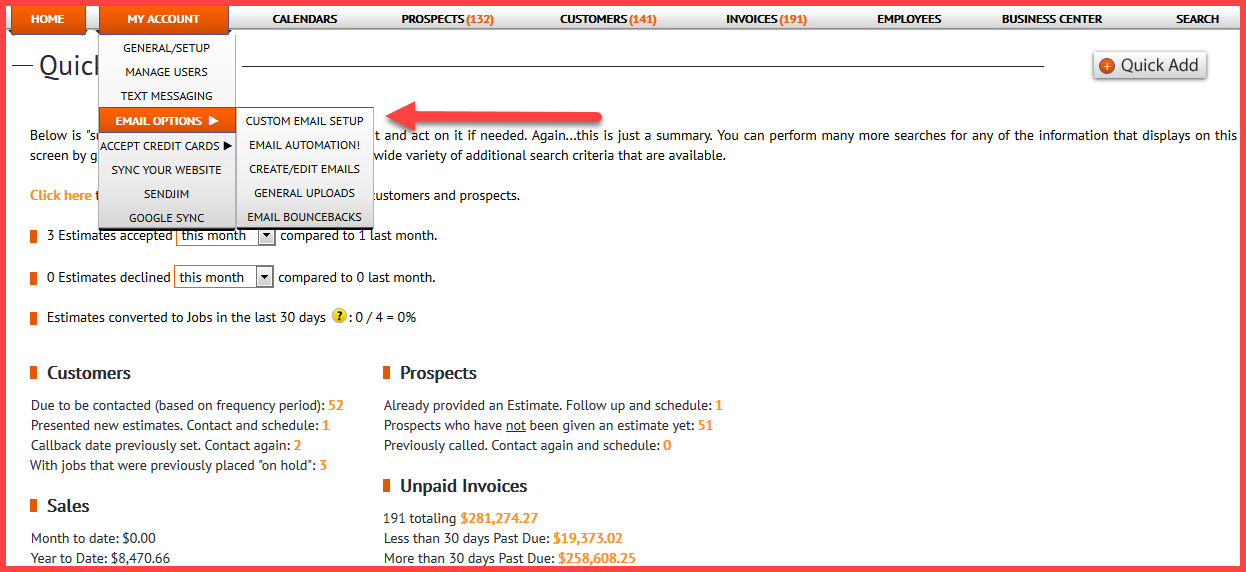A detailed screenshot captures a bustling computer interface for a website, predominantly featuring a white background with an orange navigation bar. The navigation options at the top are as follows from left to right: Home, My Account, Calendars, Prospects, Customers, Invoices, Employees, Business Center, and Search. The 'Home' tab is highlighted in orange with white lettering, while 'My Account' appears to be the selected option. Under 'My Account,' a dropdown menu displays: General/Setup, Manage Users, Text Messaging, Email Options (currently selected and highlighted in orange), Accept Credit Cards, Sync Your Website, Send, an unreadable label, and Google Sync.

Selecting 'Email Options' reveals a secondary dropdown to the right with the following selections: Custom Email Setup, Email Automation, Create/Edit Emails, General Uploads, and Email Bouncebacks. A light red arrow has been added to the image, pointing directly at 'Custom Email Setup.' Beneath this cascade of menus, a partially obscured paragraph is visible, indicating underlying content. At the bottom of the screenshot, additional tabs labeled Customers, Prospects, Sales, and Unpaid Invoices can be seen, further hinting at the website's extensive functionality.